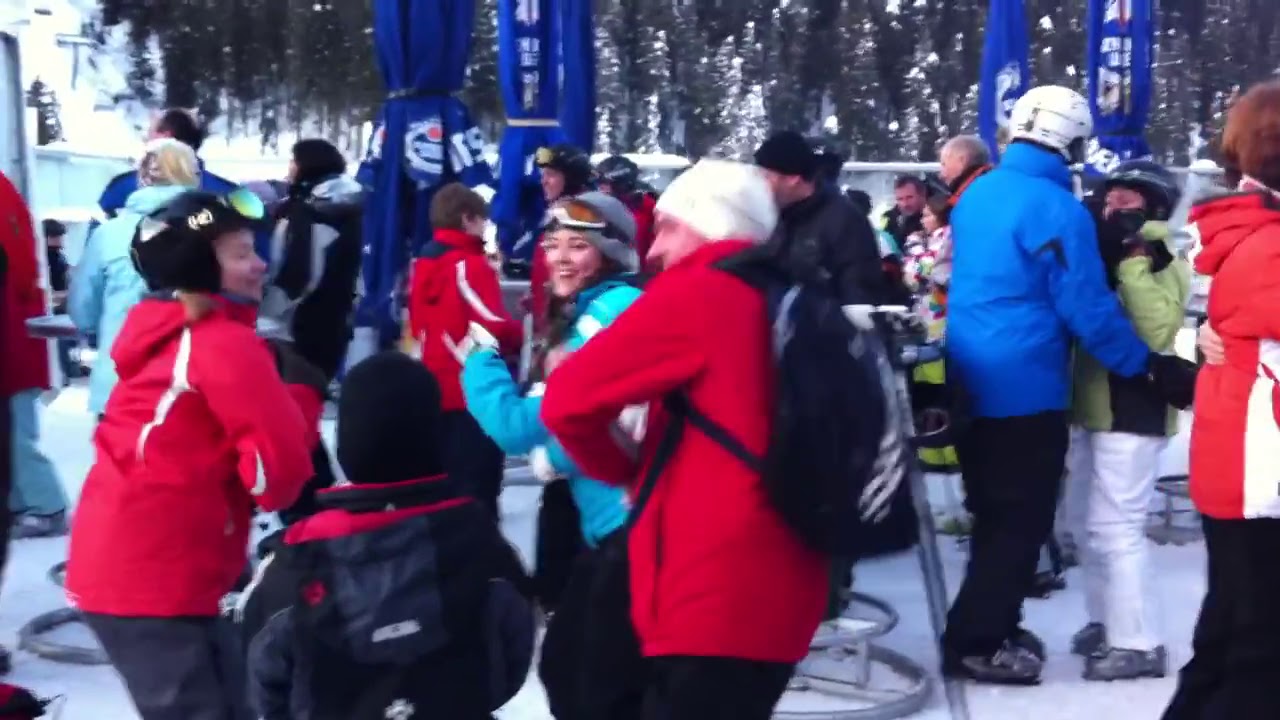The image depicts a vibrant winter scene featuring approximately 20 people gathered outdoors on a snowy surface, possibly at a ski resort. They are dressed in various types of warm outerwear, including blue and red jackets, and some are wearing helmets and ski goggles. Prominently in the center, a man in a red coat with a black backpack and a white beanie stands out, facing left. The group is primarily positioned in the center of the image, surrounded by trees laden with snow in the background. Vertical blue banners with illegible white lettering and a potential ski lift are visible in the backdrop, hinting at an organized outdoor event. Steel round wire objects and the diversity in the ski boots further contribute to the lively and detailed winter setting captured on what appears to be a cold, snowy day.